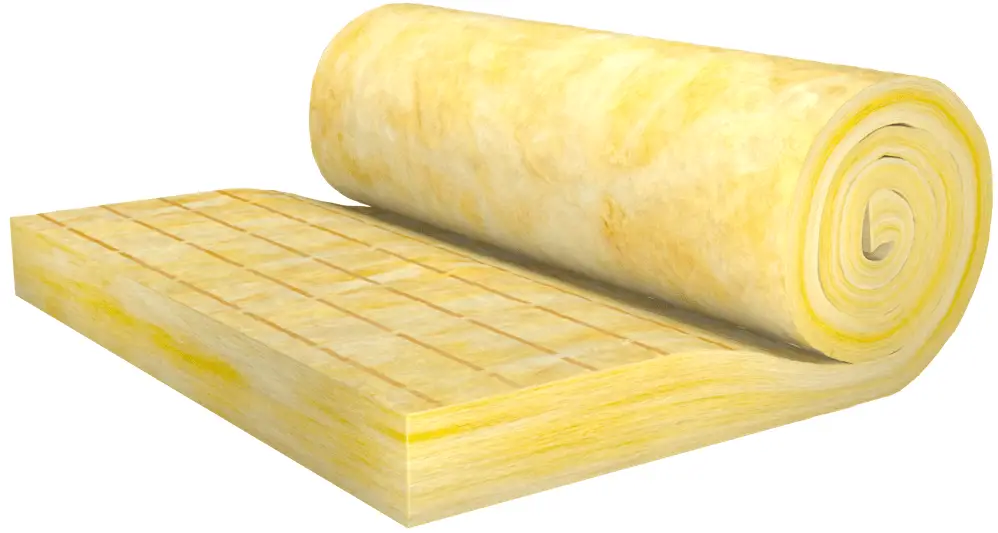The image depicts a thick roll of what appears to be yellow and white glass wool or insulation material, characterized by its soft, memory foam-like texture. The roll, which is approximately half a foot thick when uncompressed, features a distinctive yellow and white swirl design. The left side of the picture shows a portion of the glass wool unrolled, revealing a checkered pattern with lines and indentations, possibly indicating where it can be cut. The right side of the image captures the rolled-up part of the material, with tightly wound circular layers creating a dense, compact appearance. The background of the image is white, providing a stark contrast to the pale yellow hue of the insulation.